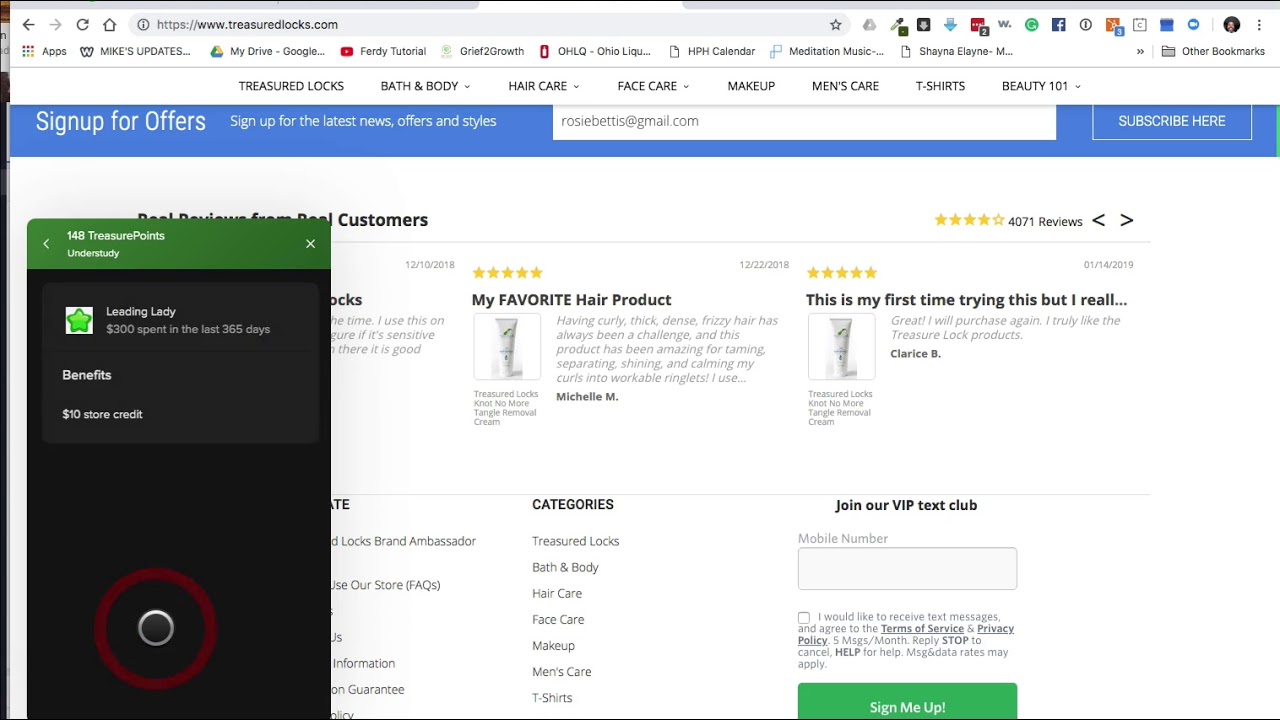This image is a screenshot taken from a web page with the URL www.treasuredlocks.com. The layout features a navigation bar with various drop-down menus labeled "Apps," "Mics Updates," "My Drive - Google," "Ferdie Tutorial," "Grief to Growth," "Ohla - Ohio Liquid," "HPH Calendar," "Meditation Music," and "Shane Shana Elaine M." 

In the center of the image, a pop-up rectangle partially blocks the content on the left side. This pop-up displays "148 Treasure Points" under a title labeled "Under Study." Below that, it reads "Leading Lady" and indicates "$300 spent in the last 365 days." Several benefits are listed, including a "$10 store card."

In the middle section of the screenshot, there are areas referencing various hair products with phrases such as "favorite hair product" and "This is my favorite first time trying this..." Additionally, there are categories and a prompt to "join our VIP text club."